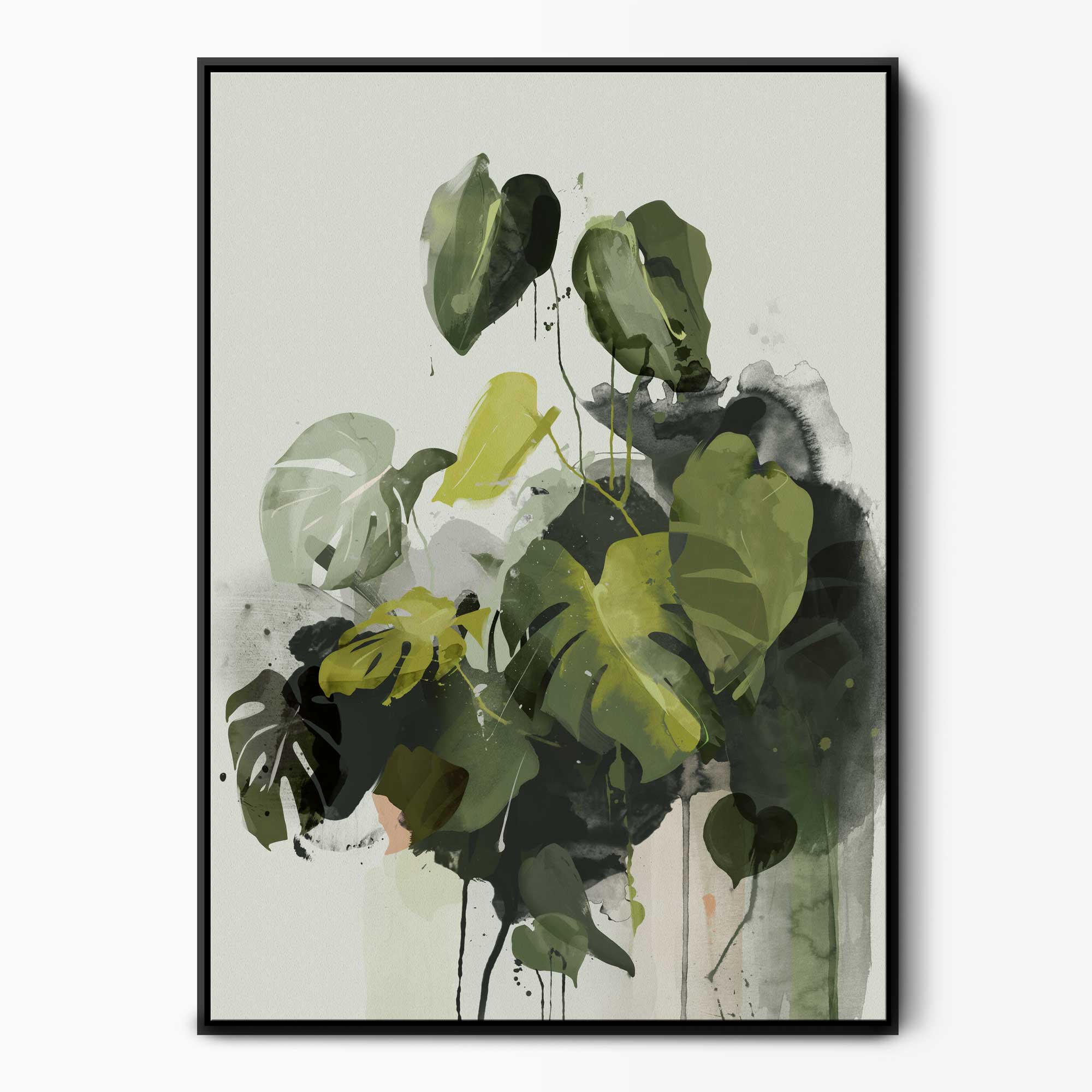This detailed image depicts a color photograph of a celebrated watercolor painting, prominently mounted on a white wall, elegantly framed by a thin black border. The painting, in a portrait orientation, showcases a lush arrangement of plant leaves cascading from the top toward the bottom. The thin, watery stems rise from a vase, merging various shades of green, including dark forest green, sage, and light green, with occasional hints of yellow and gray. The leaves vary in shape and size, with the larger, more pronounced ones at the vase's bottom giving way to smaller, uniquely shaped leaves as they ascend. Some leaves are heart-shaped, others have fingers extending outward, and the paint appears smudged, blending into subtle water stains that grace the canvas, creating an artful flowing effect. This composition captures the natural mystique of the foliage against the light greenish, almost grayish background.